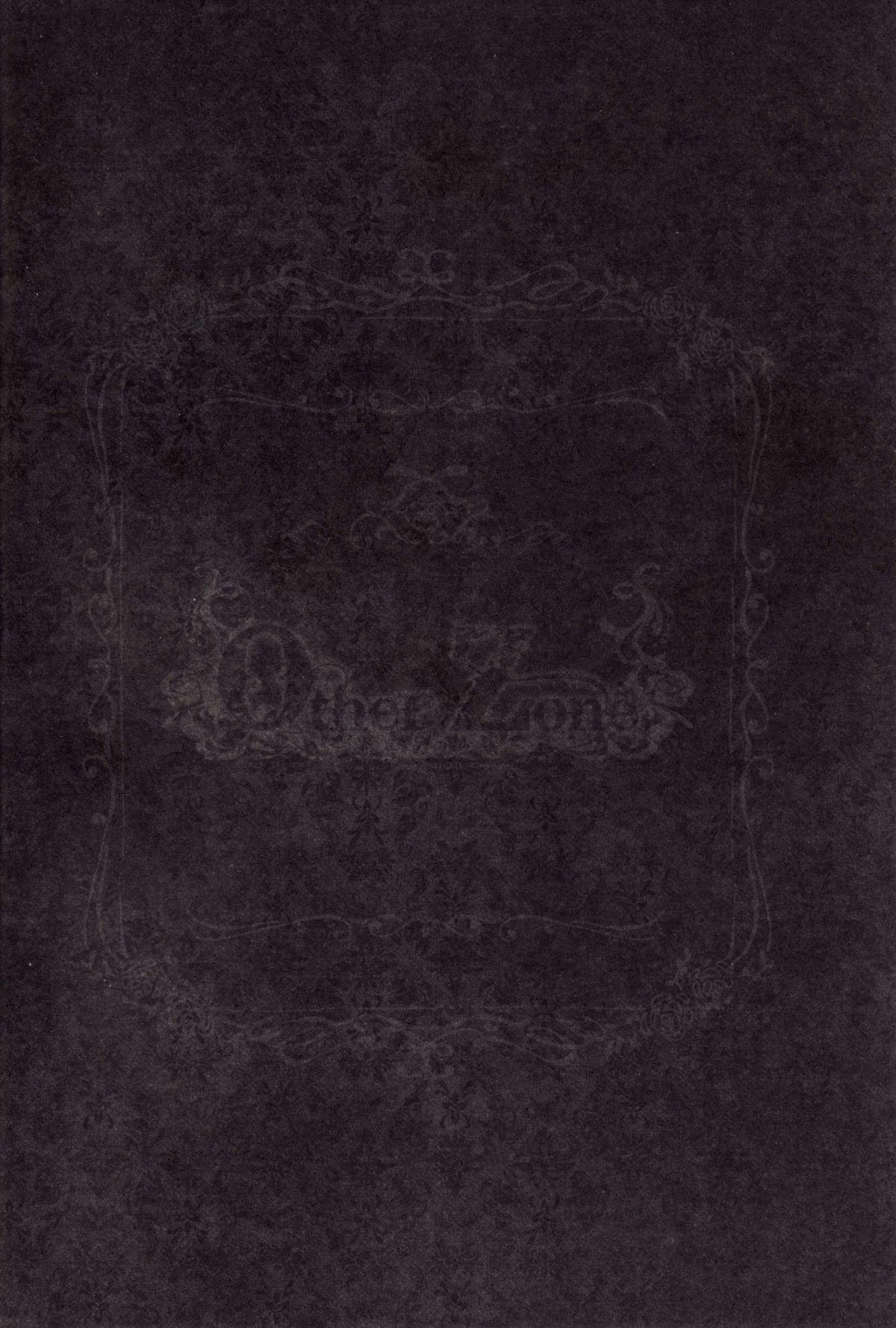This image is a very dark, vertically-oriented, rectangular photograph that resembles the texture of dark gray or light black velvet. It features subtle variations in its dark coloring, giving it a slightly patterned appearance. At the center, an ornate, square-shaped frame with rounded edges and intricate ornamental designs - reminiscent of Victorian architecture - encases the text "Other Zong," with an uppercase "O" in "Other" and an uppercase "Z" in "Zong." This text is faintly etched and almost blends into the blackness of the image, making it just barely perceptible against the dark background. The overall effect is that of an enigmatic graphic with no border frame or identifying markers, possibly evoking the sense of a mysterious webpage background or an unidentifiable material.